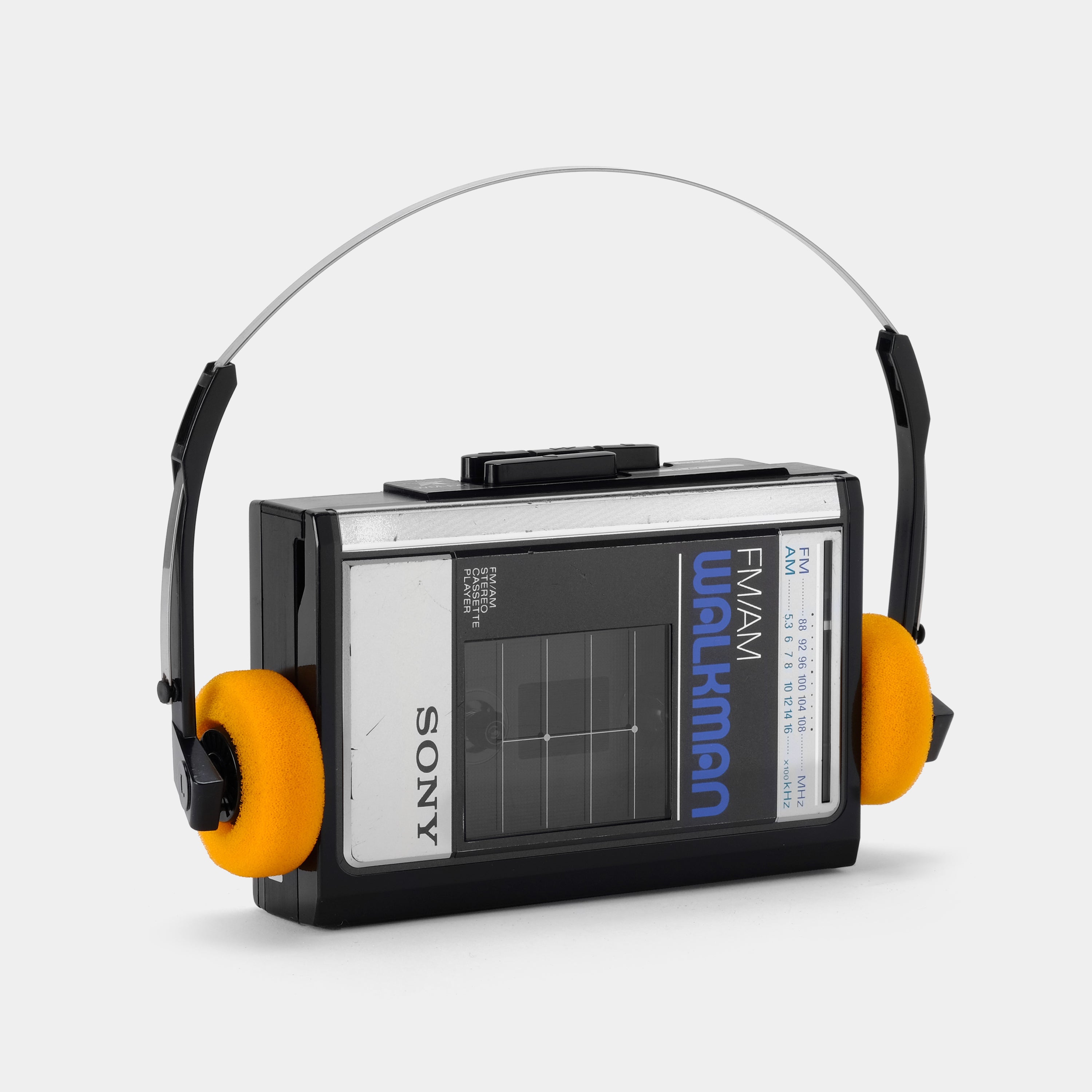This photograph captures a classic Sony Walkman from the 1980s, positioned vertically against a white background. The Walkman features a mainly black body with silver accents, including a transparent plastic window that reveals the cassette tape compartment. Dominating the center of the device is a silver panel with intricate labeling for both FM and AM radio frequencies; FM frequencies range from 88 to 108 MHz while AM frequencies range from 5.3 to 16 x 100 kHz. Just above this, in white text over a black background, it reads "FM/AM" and beneath it, in blue stylized text, is the iconic "Walkman" logo. At the top right corner, the brand name "Sony" is prominently displayed in black serif text. The device is accompanied by a pair of mustard yellow ear-pads that sit on either side of the Walkman, connected by a thin black vertical piece and a silver band. This detailed composition celebrates the nostalgic look and multifunctional features of the legendary Sony Walkman.